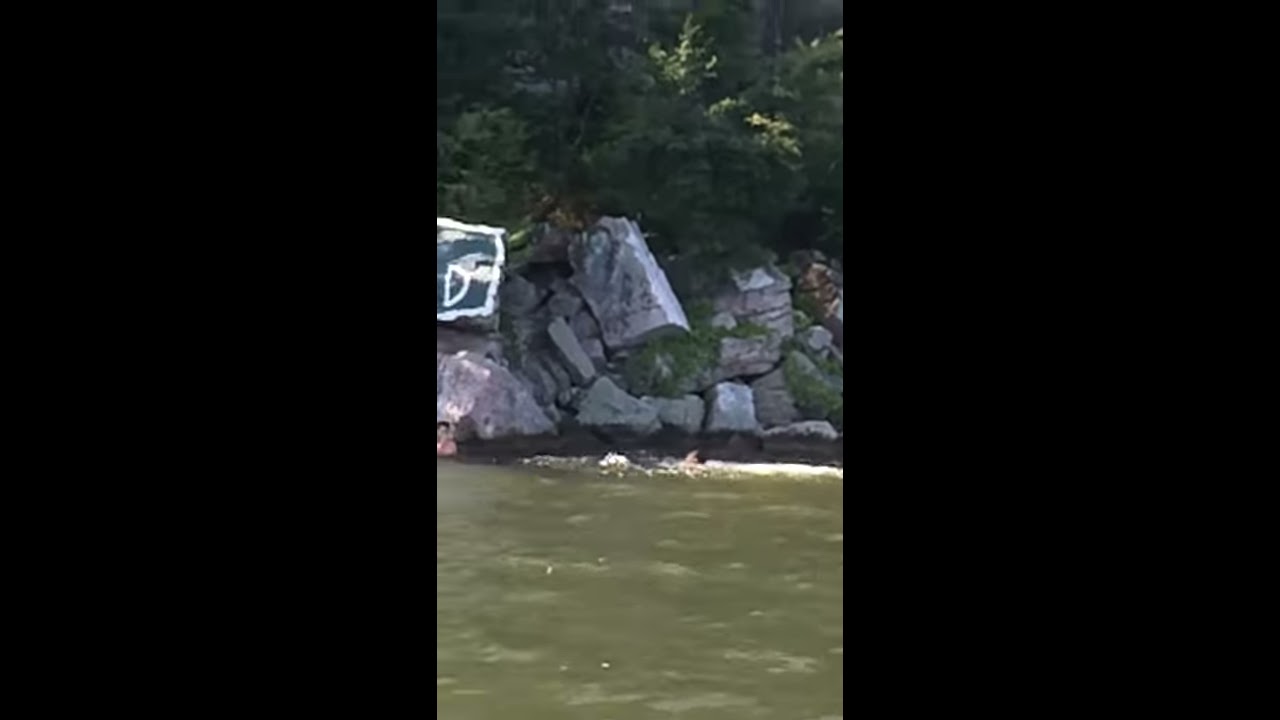The image captures a murky, dark green body of water that extends across nearly half of the frame, appearing choppy and dirty like a river or lake. Emerging from this foreboding water, you can see the heads and shoulders of two individuals: one in the center with just their head visible and another on the far left. Above the second person, there's a sign featuring the letter "D," possibly chalked onto a nearby surface or digitally added. The background transitions into a precarious, rocky hillside with large, squared-off boulders resembling massive cement blocks, some measuring three to four feet high and two feet wide. These boulders, covered in patches of moss and sparse vegetation, form an unstable boundary between the water and a dense forest of dark, green trees that loom above. The entire scene is framed by wide black borders on both sides, intensifying the dark, foreboding atmosphere of the image.